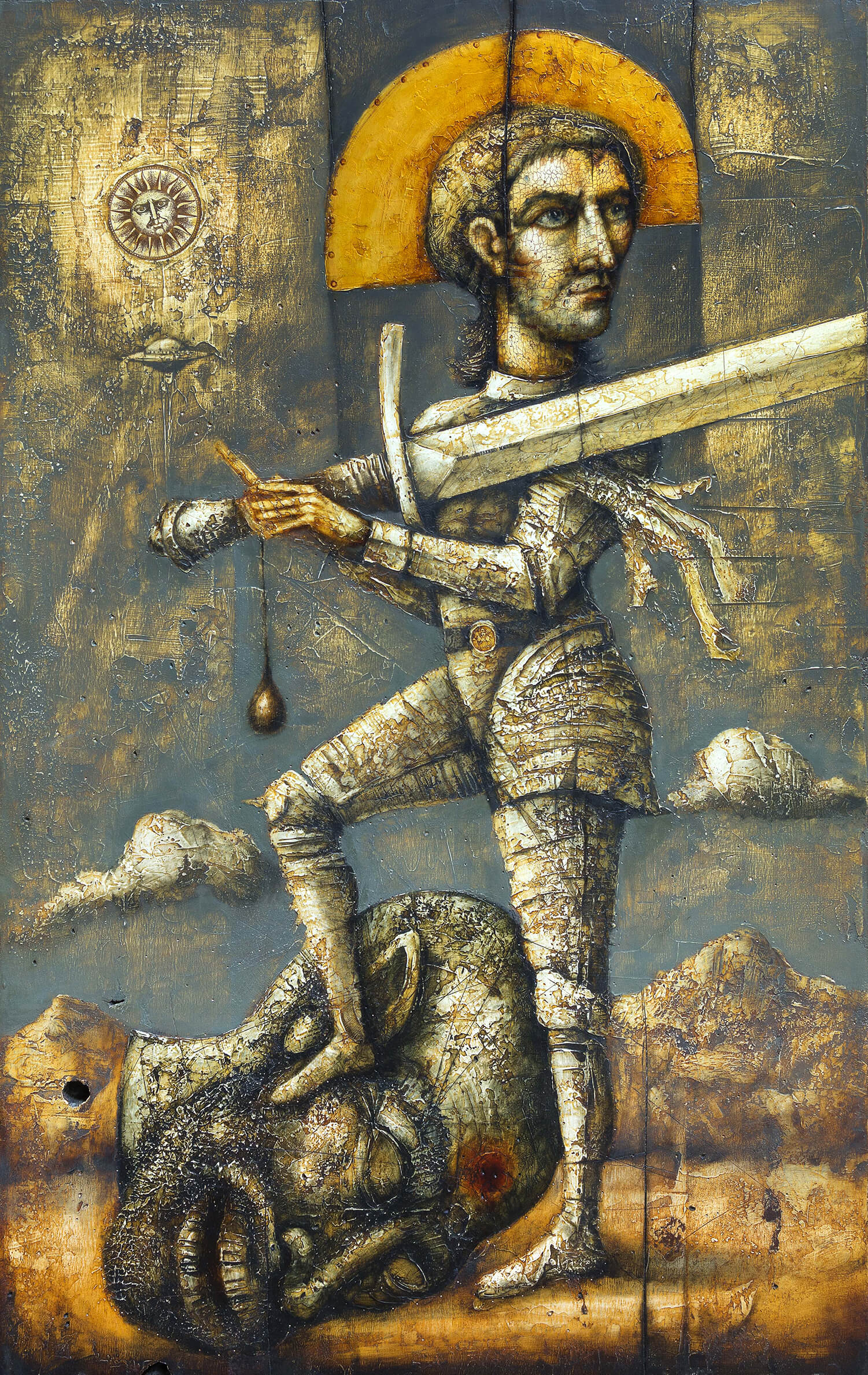This detailed painting, tall and rectangular in shape, features a rich and complex scene against a greenish-gray and black background adorned with various designs. On the left side near the top, there's a gold sun design, below which a planet design can be seen. Central to the composition is a man dressed in a silver knight's costume, resembling medieval armor. He wears a gold semicircle hat that could be interpreted as a halo and has long, dirty hair and a prominent nose. The man, who appears to be of European descent, gazes to the right, gripping a large broadsword in his left hand that points to the same direction. His right foot rests assertively on the severed head of what could be identified as a giant or a demon, located in the bottom left corner of the painting. The head, with an open mouth and downcast eyes, is adorned with a beard. The background features an intricate and vibrant mix of brown and white mountains, a blue sky, and puffy white clouds. Intriguingly, just below the gold sun, there is a depiction of a UFO or an alien spaceship. This painting vividly combines elements of myth and history with fantastical features, creating an engaging visual narrative.